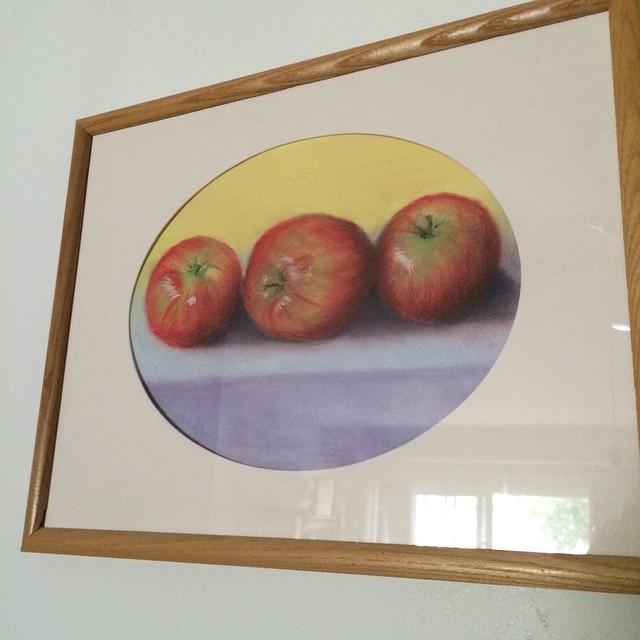A photograph captures a hand-drawn artwork of three apples, framed and hanging on a wall in a home. The frame is made of light brown wood, and a light beige mat with a circular cutout surrounds the drawing. The apples in the artwork are primarily red with hints of green and yellow, depicting a ripe and natural look. They rest on a light blue or purplish surface, with a yellow background above them. The light in the drawing appears to come from the top left-hand corner, casting subtle shadows. The glass covering the frame reflects a window or French door behind the photographer, through which a green tree is visible, adding a sense of depth and context to the setting.